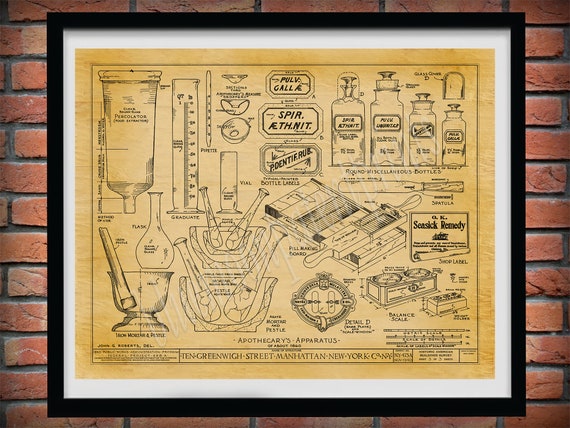This photograph captures a framed and matted antique poster, meticulously mounted on a classic red brick wall. The poster itself is an old-fashioned, slightly yellowed beige piece of paper encased in a black frame with a white matting accentuating its vintage appeal. Dominated by an array of sepia-toned illustrations, the poster serves as a detailed diagram for apothecary apparatus. The assortment of images includes various glass bottles, mortars, and pestles, alongside intricate machinery potentially linked to the distillation of spirits or moonshine. Each illustration is accompanied by descriptive captions, hinting at their use. Notably, at the bottom of the poster, it prominently declares "Apothecary Apparatus" followed by the address, "10 Greenwich Street, Manhattan, New York," framed within a slender rectangle. The careful placement and detailed imagery make this piece a rich tapestry of scientific and historical intrigue.